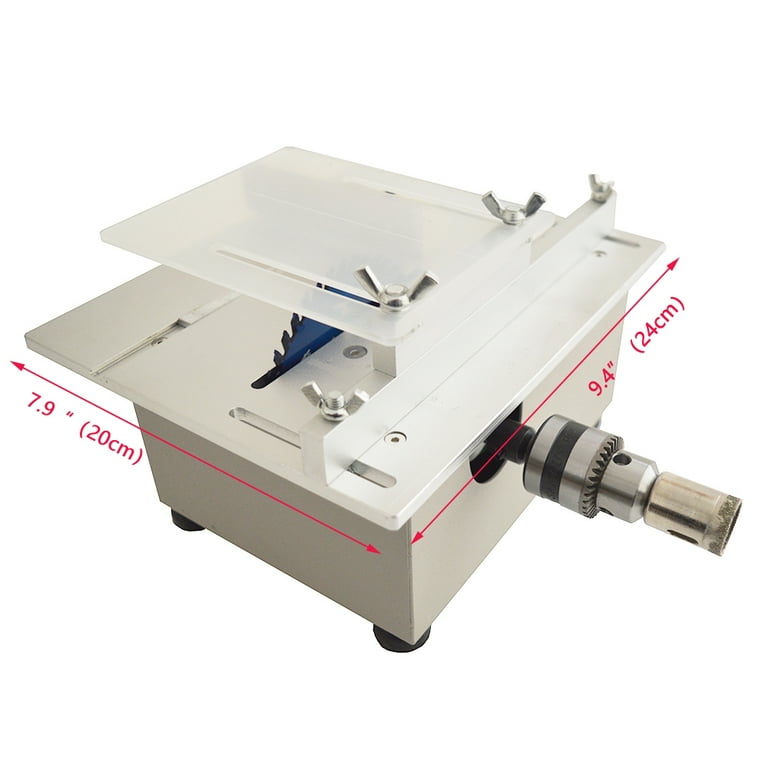The image depicts a mechanical table saw set against a white background. The base of the saw is mostly gray with a tan hue, while the top part is white. Central to the design is a metal saw blade protruding from a small black opening in the middle. The top of the saw blade is secured by a clear plastic cover fastened with chrome wingnut screws. Additionally, there is a cylindrical metal object extending from one side of the saw. On the sides, the saw features measurement markings: the left side displays "7.9 inches, 20 centimeters" and the right side "9.4 inches, 24 centimeters." The machine is stabilized by small black knobs, likely positioned at each corner for additional support.